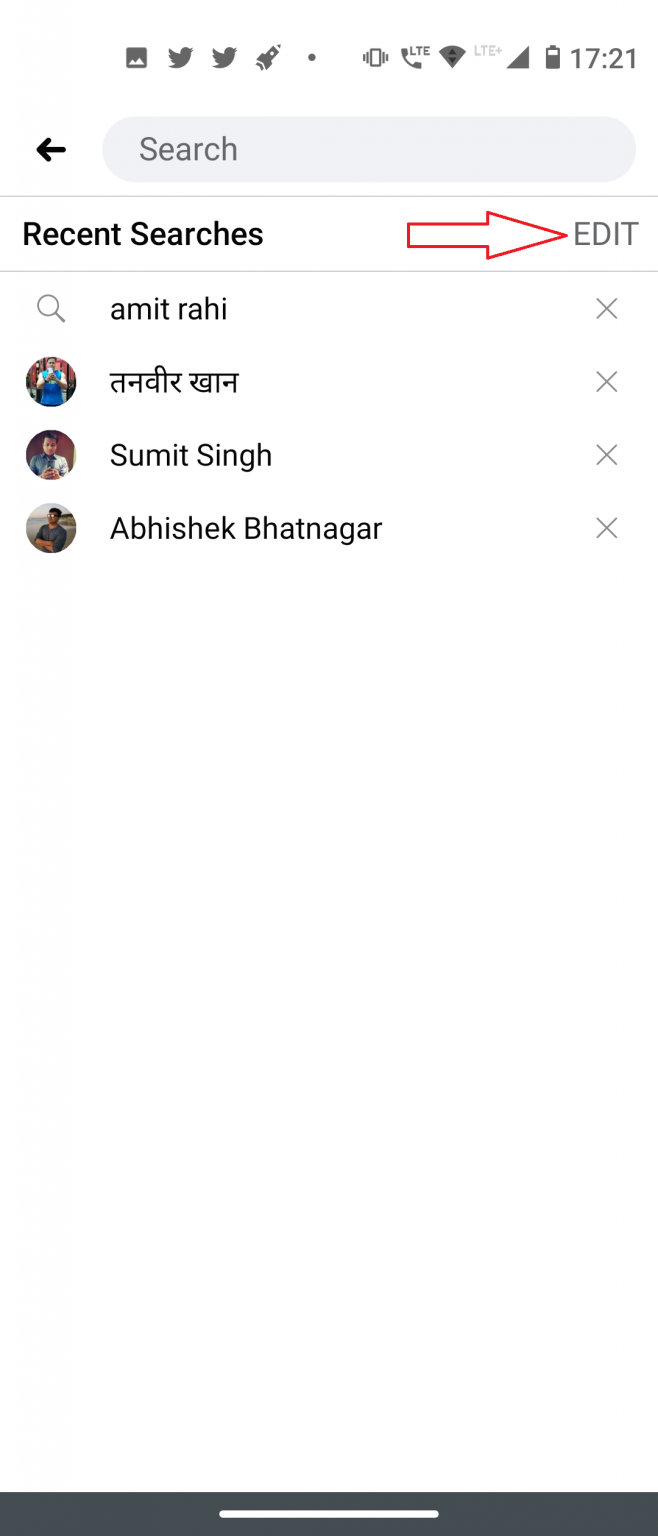This image captures a screen from an unspecified app displaying a 'Recent Searches' page. The primary content includes a list of recent searches with names such as "Amit Rahi" (A-M-I-T R-A-H-I), "Sumit Singh" (S-U-M-I-T S-I-N-G-H), and another name in an Indian language. There is also a name in an Indian language script. At the top of the screen, a search bar is present with an adjacent back button and a distinctive white arrow with a red outline pointing to the word 'edit,' suggesting functionality for possibly removing or editing search entries. Each search entry features an 'X' allowing users to delete them from history. The screen's background is plain white with all text in black, and most of the page is occupied by blank space. Additional elements visible include the user's notification area containing a few Twitter notifications, indicating the device is set to Vibrate mode, and a recent screenshot. The overall context or purpose of the app remains unclear.